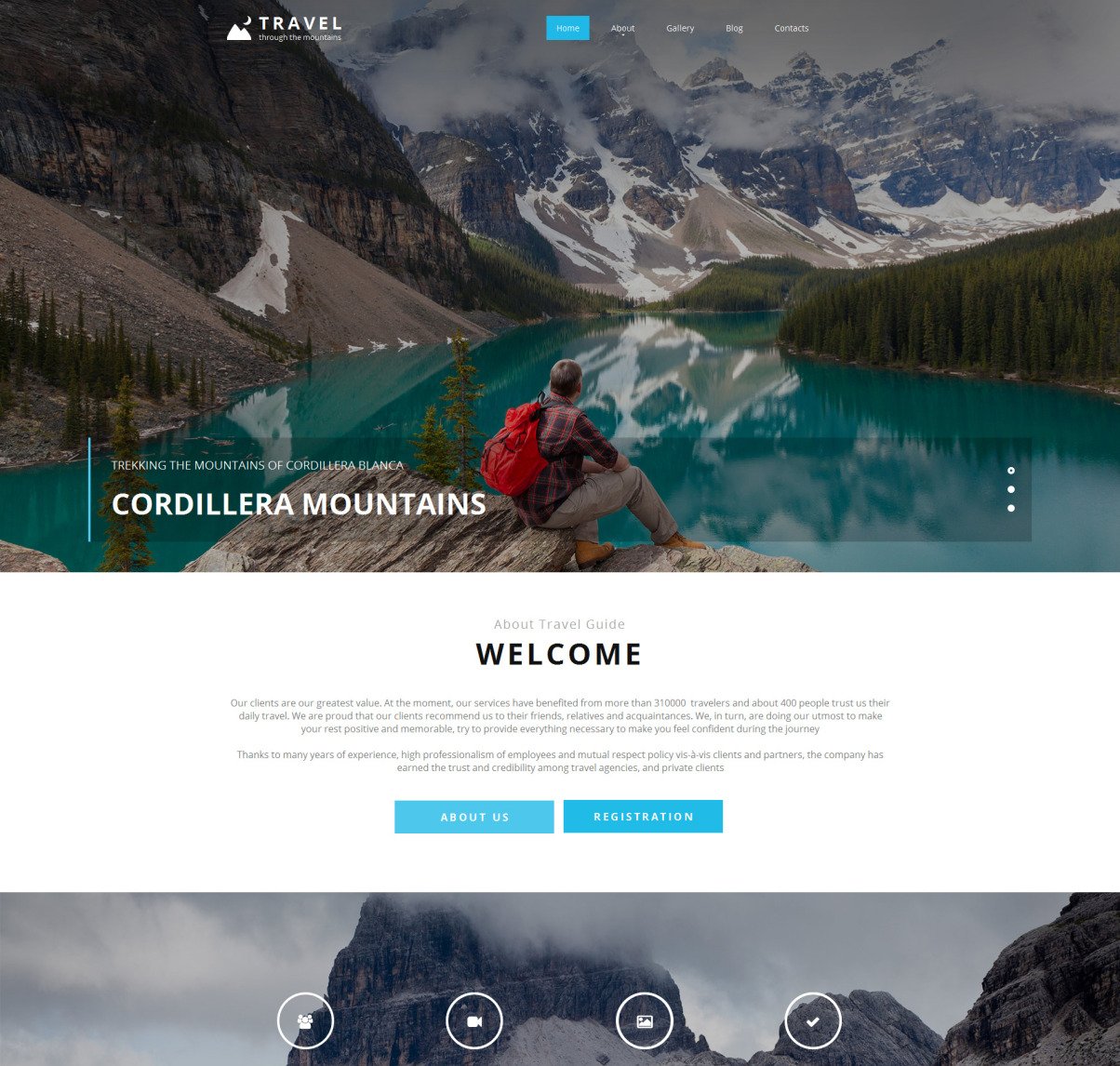A dynamic travel website featuring a prominent stock image of a male hiker gazing from atop a cliff at the expansive landscape below, which includes a lake, mountain ranges, forests, and snow-capped peaks, known as the Cordillera Blanca Mountains. The image is overlaid with the label "Trekking the Mountains of Cordillera Blanca." Superimposed on this breathtaking backdrop is the website navigation, including links to the homepage, about page, gallery page, blog page, and contacts page.

A welcome note introduces the site's ethos, emphasizing that clients are its greatest asset. It proudly states that their services have been enjoyed by over 300,000 travelers and trusted by around 400 individuals daily, with many clients recommending the site to their friends, relatives, and acquaintances.

Beneath the welcome note are buttons for "About" and "Registration." Near the bottom of the page are four distinctive icons: a check mark symbolizing reliability, a gallery icon offering access to travel photos, a camera icon likely linked to user-uploaded content, and a community or group icon representing the site's vibrant user community.